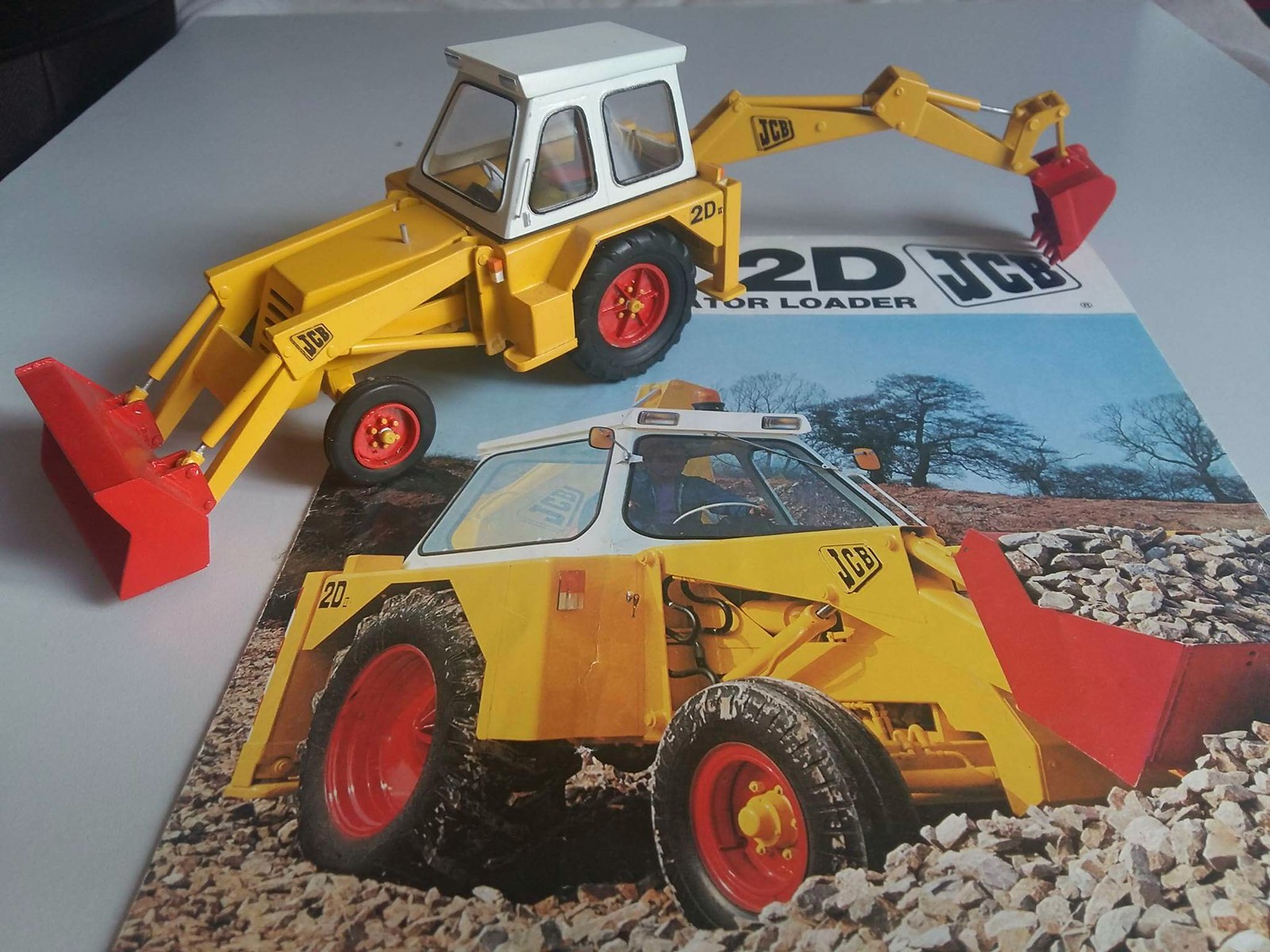The wide rectangular image showcases a detailed model of a construction vehicle placed on a glossy white table. The table surface is visible at the top left and right corners. The model, a replica of a front loader or tractor loader, features a large red scoop in front and a smaller red scooper mechanism at the back. The construction vehicle itself is painted in bright yellow with a white roof, black tires, and red rims. This model is positioned on top of a large paper that appears to be from a magazine or manual, largely covering the bottom of the image and tapering towards the top. The magazine features an action shot of the full-sized construction vehicle in a rock quarry, highlighting its functionality of shoveling rocks. The overall presentation emphasizes the details and design of both the miniature model and its real-life counterpart, with branding references such as "JCB" and partial text indicating "something 2D" possibly related to the loader’s name or model.